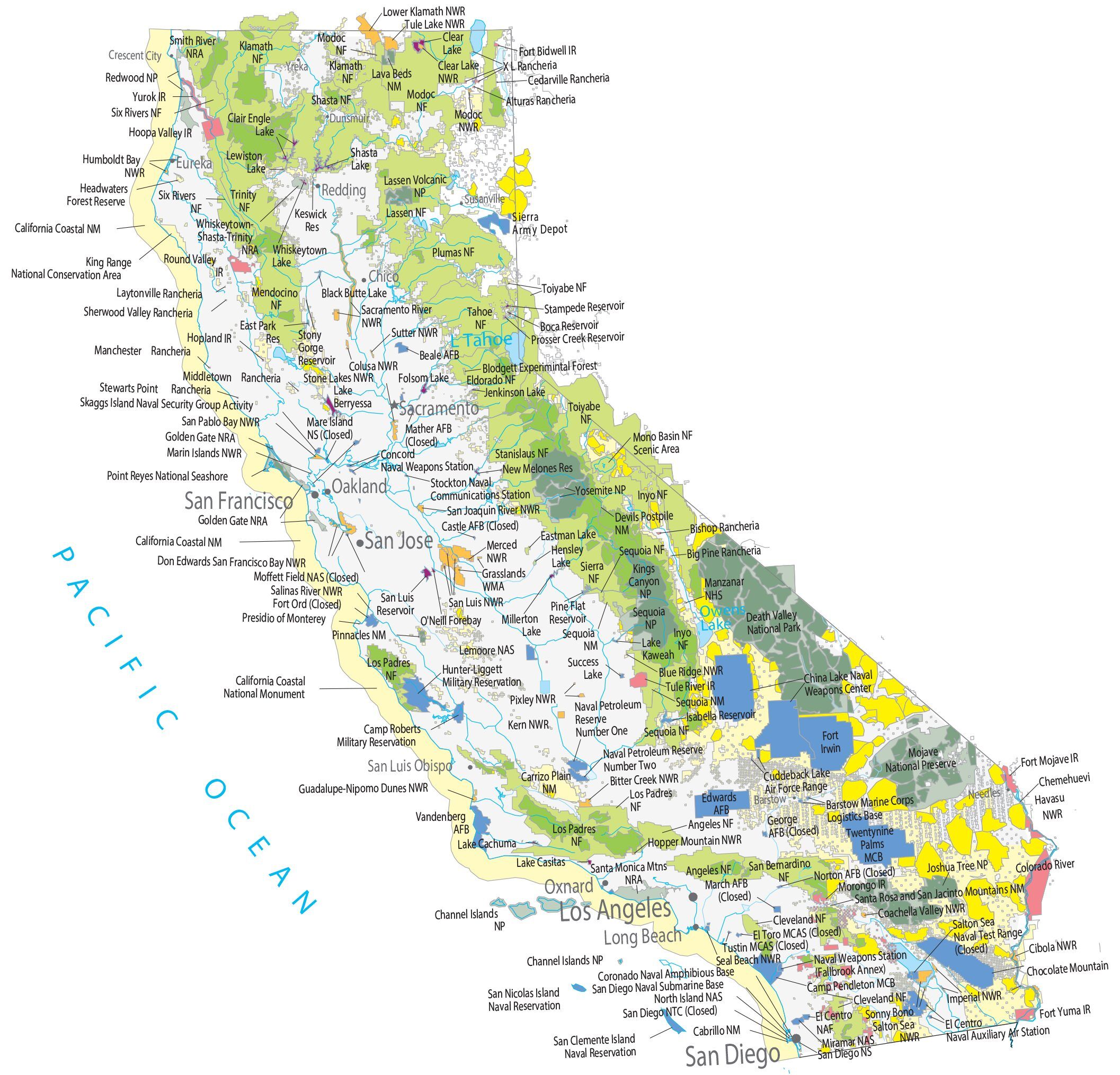This detailed color illustration is a topographical map of California, extending from the northern border to the southern border. The Pacific Ocean, labeled in blue text, is situated to the west. The map features a variety of shaded areas - light to dark green hues represent different terrains, and there are additional bluish and gray regions, particularly in Southern California. The mountainous areas are depicted in lime green, while lower elevations are in a cream color, and the Central Valley stands out in white. Although the map does not include a key to explain the colors, it is populated with black text indicating both major cities and smaller locales, such as Oakland, San Francisco, Sacramento, Eureka, and Redding. Various rivers and lakes, like Eastman Lake and Hensley Lake, are also marked, along with points of interest including the Sierra Nevada and Pine Flat Reservoir. The map omits neighboring states but provides a comprehensive topographical and geographical overview of California.